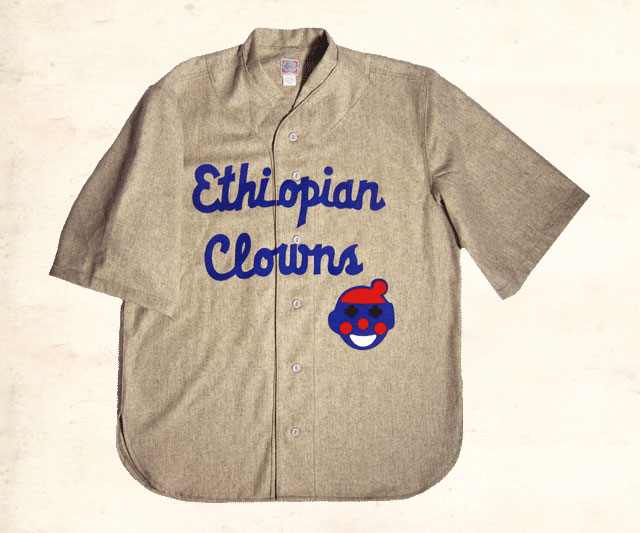This is a square color photograph of a vintage baseball jersey, set against a background that resembles an aged piece of paper in beige with brown stains. The jersey itself is a light gray button-down shirt with a slight collar, appearing unused and recently ironed. It features light brown buttons and a visible tag at the back of the top. Emblazoned across the chest in big blue cursive letters, it reads "Ethiopian Clowns," with "Ethiopian" positioned above "Clowns." To the lower right of this text, if looking at the jersey, there is an image of a clown head adorned with a red hat topped by a pom-pom. The clown's face is blue, with two black crosses for eyes, a red dot for a nose, and red dots for cheeks. The smiley face is colored white, creating a vivid contrast against the gray material of the jersey.